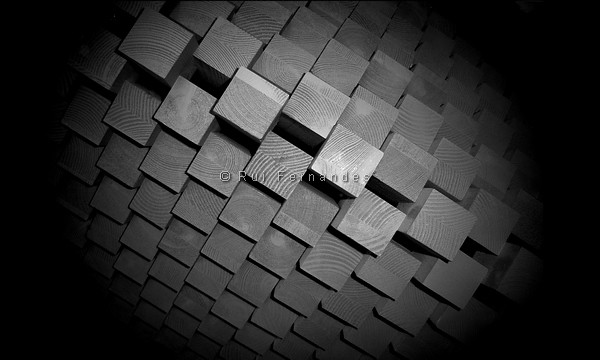This horizontally aligned rectangular image, potentially computer-generated and monochrome, features a striking centerpiece against a solid black background. Dominating the center is a complex, almost football-shaped structure composed of numerous small, gray squares with subtle swirled patterns, possibly resembling wood grain. These squares, or wooden blocks, are arranged in a symmetrical and linear geometric pattern, some of which are raised, creating subtle gaps between adjacent squares. The overall object appears three-dimensional, as if viewed from above, showcasing the tops of these blocks. Central to this intricate pattern is a barely discernible watermark in small gray text that reads "© Rui Fernandes," blending into the grayscale tones of the image.